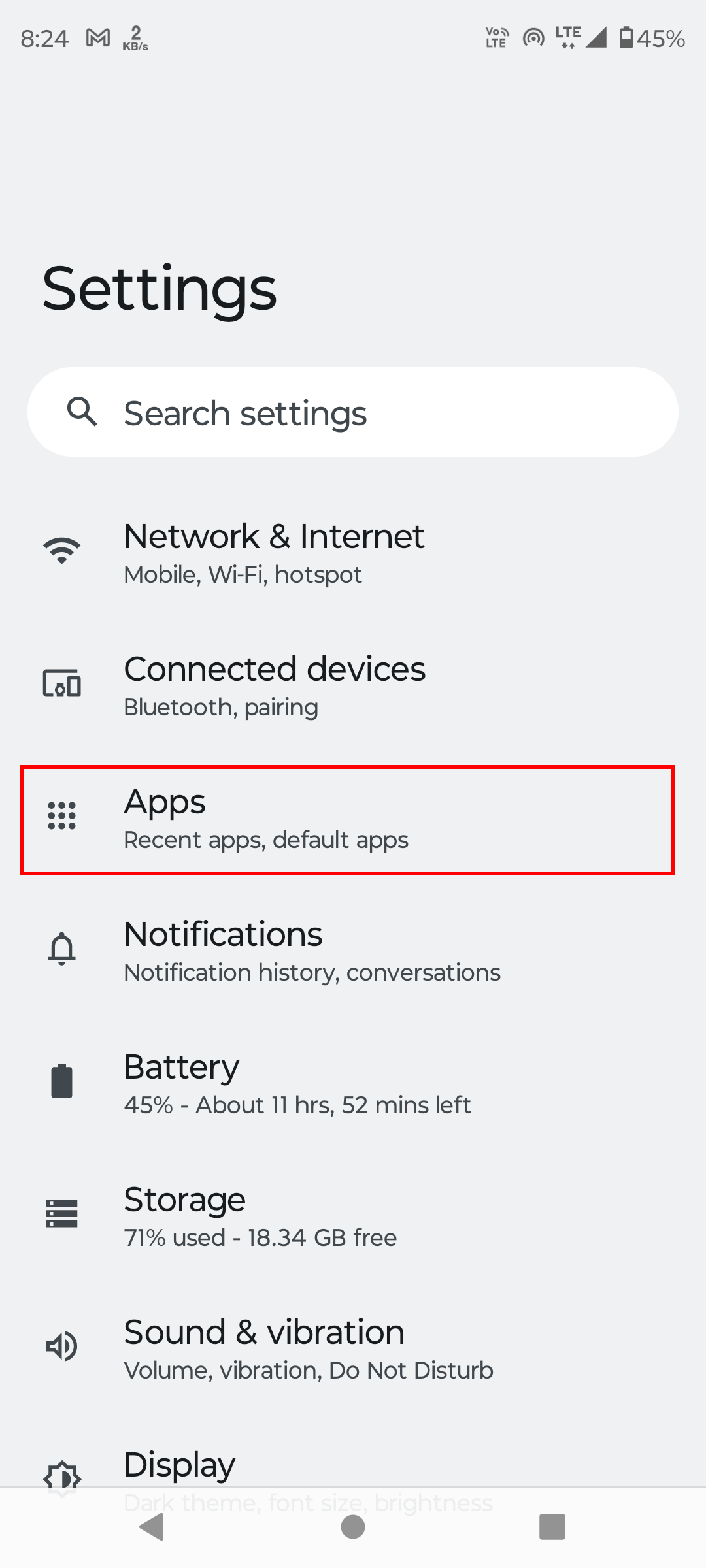This image is a vertically oriented screenshot taken from a smartphone. The background is a uniform medium gray with no texture or gradient. 

In the top left corner, the time is displayed as 8:24, and there are icons indicating a mobile network signal (M) and data transfer rate (2 KB/s). On the top right, the status bar shows the LTE signal, Wi-Fi connection, a sideways triangle (possibly indicating a VPN or data saver), and the battery life at 45%. 

The main content of the screen is the settings menu, with the word "Settings" prominently displayed in bold black letters at the top. Below this is a white search bar labeled "Search settings."

The settings menu options listed include:

- **Network & Internet** with an accompanying icon, detailing mobile Wi-Fi, hotspot, etc.
- **Connected Devices** with icons for Bluetooth and pairing.
- **Apps** with a red box highlighting areas for recent apps and default apps.
- **Notifications** with a bell icon, showing notification history and conversation settings.
- **Battery** with an icon indicating 45% charge and an estimated 11 hours and 52 minutes of remaining battery life.
- **Storage** with an icon showing 71% used and 18.34 gigabytes free.
- **Sound & Vibration** with icons for volume, vibration, and do not disturb settings.
- **Display**, partially visible, indicating settings for screen display.

The bottom of the screen is partially obscured by the navigation bar, which has the traditional Android icons for back (triangle), home (circle), and recent apps (square).